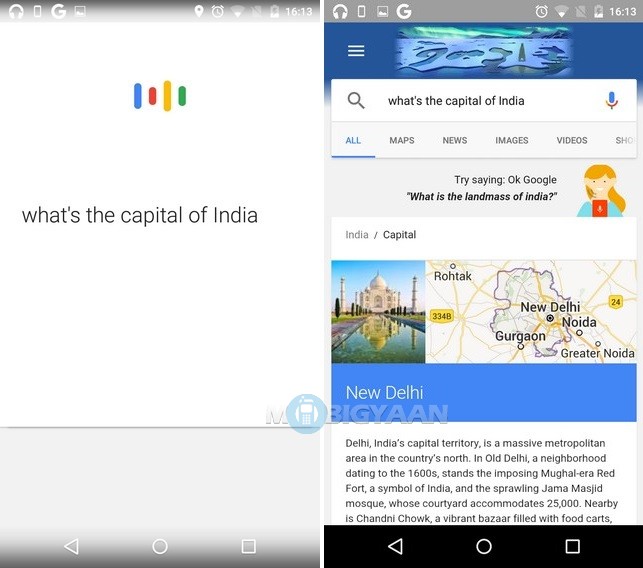The image displays two side-by-side screenshots overlaid with a business logo purportedly named "Moe Big Yon." The logo features the text "MEIGYAAN," where the second 'O' is substituted with a blue phone symbol encased in a blue thick circle. Both screenshots are taken on the same Android device, as indicated by their identical top toolbars which display icons for headphones, a rectangular phone, a photo, Google, location, clock (showing 16:13), Wi-Fi, a page with a slash through it, and battery status. Additionally, both screenshots feature the standard Android navigational buttons—a back arrow, a circle, and a square—at the bottom.

The left screenshot captures a user asking Google Assistant, "What's the capital of India?" The right screenshot shows the response from Google Assistant, displaying a Google search result that succinctly identifies "New Delhi" as the capital of India.